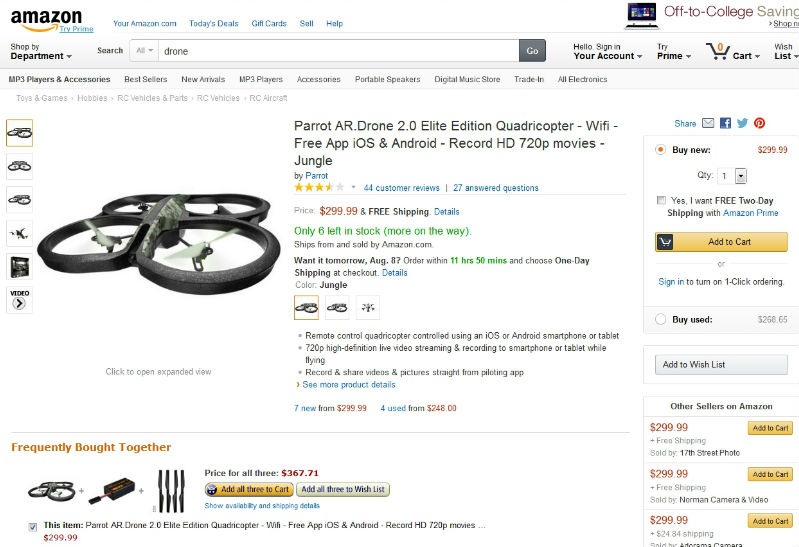**Detailed Caption:**

In this image, we have a detailed screenshot of an Amazon product page primarily featuring a white background with various text and buttons. At the very top left, the iconic Amazon logo is prominently displayed, accompanied by a call to action, "Try Amazon Prime." Moving right, a series of navigational links appear, including "Your amazon.com," "Today's Deals," "Gift Cards," "Sell," and "Help." Further to the right, there is a small advertisement featuring a computer and the message "Off to College Savings - Shop Now."

Directly below this, a navigation bar allows users to shop by department. In this particular instance, the search bar contains the word "drone," and a "Go" button is positioned to the right. Additional options such as "Hello, Sign in to your account," "Try Prime," "0 Items in Cart," and "Wishlist" are also present in this section.

Proceeding downward, the user is presented with more navigational options. This includes selectable text categories like "MP3 Players and Accessories," "Bestsellers," "New Arrivals," "MP3 Players," "Accessories," "Portable Speakers," "Digital Music Store," and "Trade-In Electronics." The specific category selected here is "Toys and Games," focused on "Hobbies," "RC Vehicles & Parts," "RC Vehicles," and "RC Aircraft."

On the left-hand side of the page, there is a large image showcasing an aerial drone, flanked by several smaller, selectable images offering various angles of the same product. The main text specifies the item as the "Parrot AR Drone 2.0 Elite Edition Quadrocopter - Wi-Fi, Free App, iOS and Android." Further details include the ability to record HD 720p movies. The item is named "Jungle by Parrot," with an endorsement of 44 customer reviews and 27 answered questions. The price is listed at $299.99 with free shipping, noting only six units left in stock and more on the way, shipped and sold by Amazon.com. There’s also a prompt for expedited delivery: "Want it tomorrow, August 8th? Order within the next 11 hours and 15 minutes and choose One-Day Shipping at checkout."

The product description highlights key features, such as remote control via an iOS or Android smartphone or tablet, 720p HD live video streaming and recording, and the ability to record and share videos and pictures directly from the piloting app.

On the right side of the screen, the buying area details the price of $299.99 with a quantity selector, a note encouraging users to get free two-day shipping with Amazon Prime, and an "Add to Cart" button. Options for "One-Click Ordering," "Buy Used," and adding items to the "Wishlist" are also visible. Additionally, other offerings for the same item and recommended accessories are displayed at the bottom left of the page.